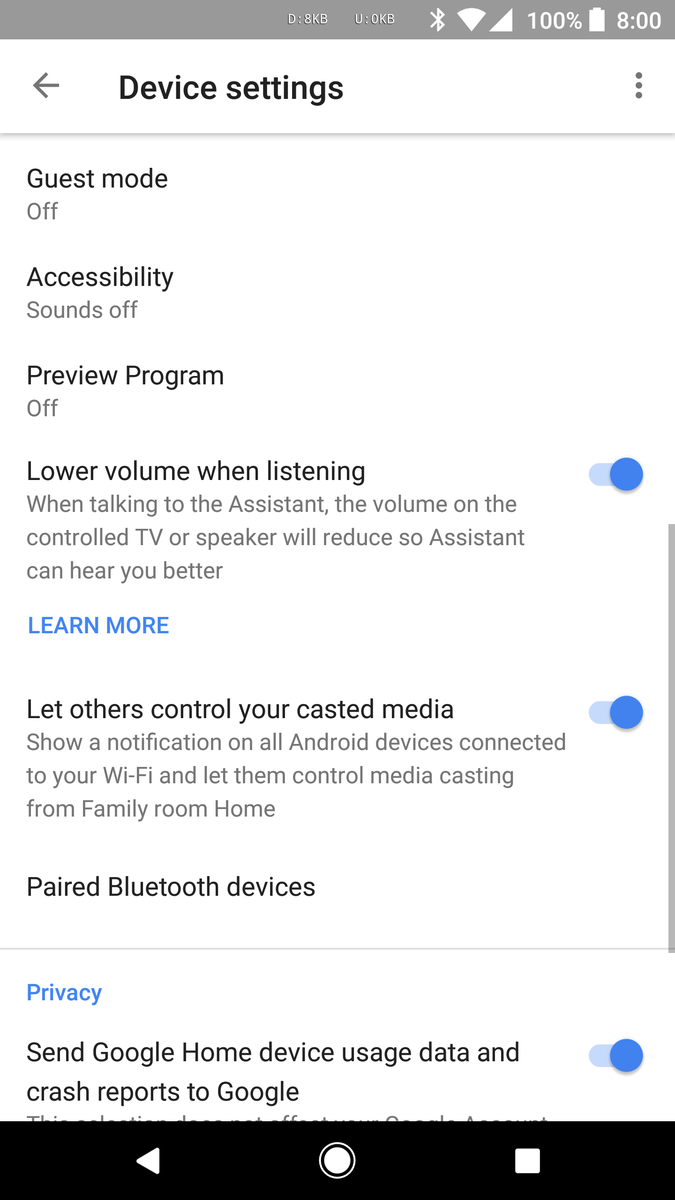Caption: 

A cell phone screen displays the settings menu, showcasing a variety of device configurations. The screen indicates a strong cellular signal, Wi-Fi connectivity, and a fully charged battery. The exact time is ambiguous, as it shows only "8:00," without specifying AM or PM. The settings currently active include "Guest mode off," "Accessibility sounds off," "Preview program off," and "Lower volume when listening." Additionally, a feature reducing volume on a TV or speaker to improve voice assistant recognition is toggled on. 

Highlighted in blue is an option to "Learn more" and settings allowing others to control cast media via notification on connected Android devices. This option is also enabled. Further details include "Paired Bluetooth devices," privacy settings sending usage data and crash reports to Google, all of which are switched on. The screen's theme features a mix of gray, white, black, and blue elements, with actionable links and enabled settings marked in blue. 

At the bottom, there is a navigation bar with icons: a white circle for the home button and a square for recent apps, with more options available upon scrolling. The top gray bar houses various phone status icons. Every visual cue and toggle setting provides a meticulous representation of the user's device settings configuration.